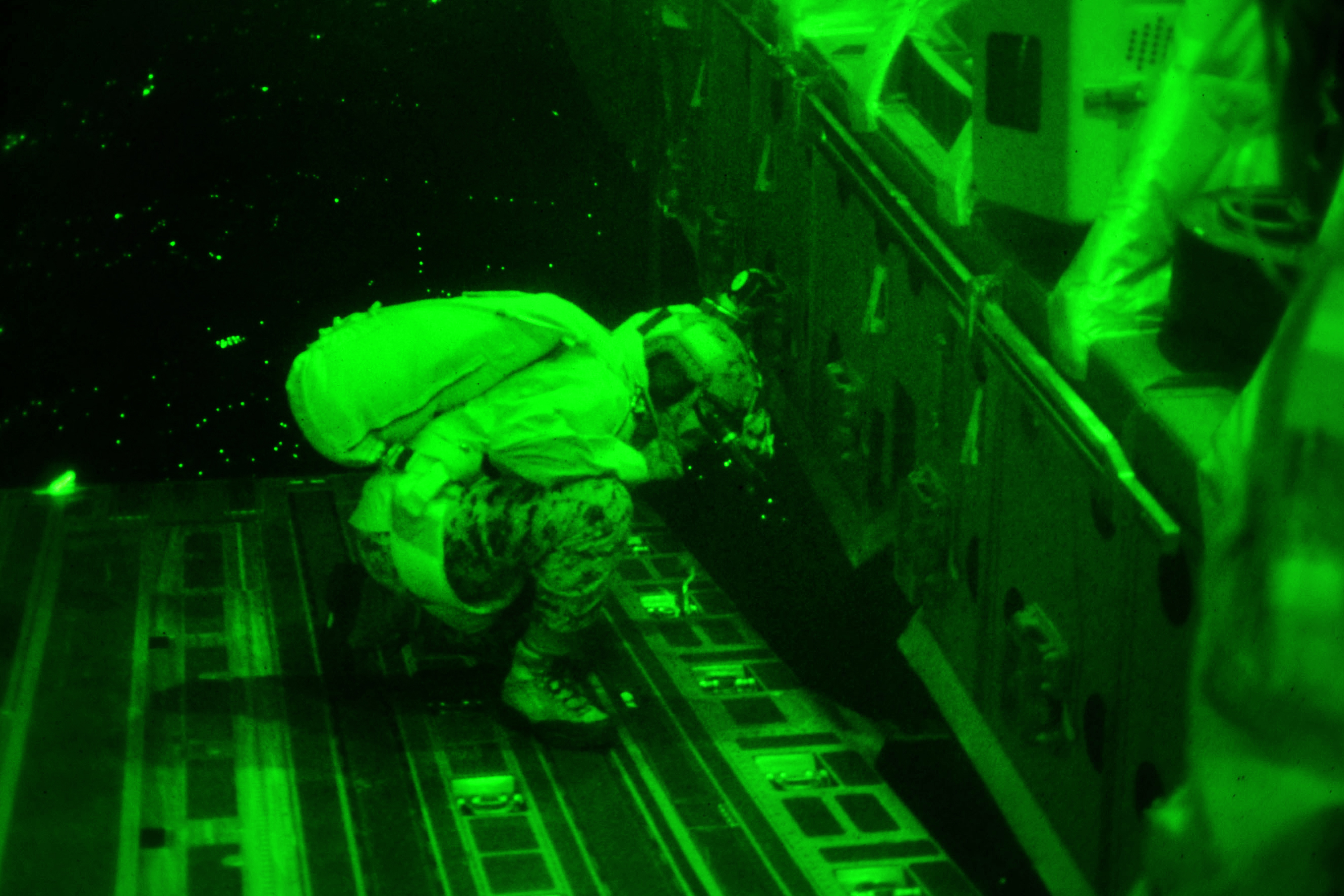This captivating night vision photograph vividly captures a dramatic scene bathed in hues of green and black, characteristic of such imaging technology. At the heart of the image, a figure dressed in a full hazmat suit and a helmet crouches on a platform. This individual, possibly a scientist or military personnel, is seen carrying a large bag or backpack, their boots planted firmly on the surface. To the right of this figure, another platform or workbench emerges from the shadows, cluttered with an old-style CRT computer monitor, various tools, and potentially some cabinets.

The setting remains ambiguous, evoking images of either a laboratory or the rear ramp of a military aircraft, such as a C-130, where personnel might prepare for a parachute jump. The background is almost entirely obscured in near-total blackness, punctuated only by occasional greenish dots that could suggest distant stars or lights. This obscured backdrop and the limited visibility enhance the mysterious and intense atmosphere of the scene.